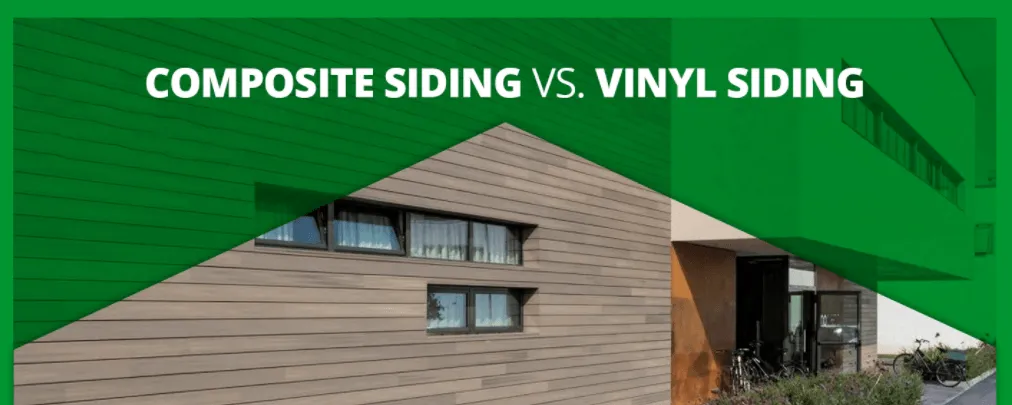This detailed, cohesive caption merges and refines the various descriptions:

"This rectangular landscape advertisement, roughly 2.5 times wider than it is high, showcases a comparison between 'Composite Siding vs. Vinyl Siding'. The bold white text, except for the thin 'VS.' in the center, is placed against a bright green backdrop that dominates about 80% of the image with a translucent triangle peak at the top. Behind this green overlay, two buildings are visible. The left building, a light brownish-gray structure with composite siding, features six small rectangular windows arranged in two rows. The right building, which has a concrete-like appearance, includes a white overhanging section with windows and an open entry door beneath. In front of this entry are three or four bicycles and some shrubbery. The scene is set against a clear white sky."